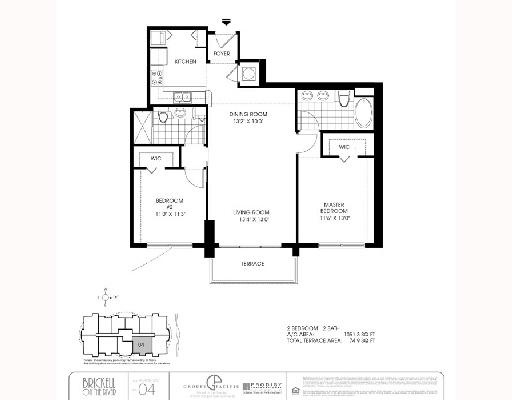This photo showcases a sketch of a floor plan, although the picture quality is notably poor, making it difficult to discern the finer details. The sketch appears to depict an apartment layout. Positioned at the bottom of the image, there is a partially legible brand name, which seems to read "Brickell on the River" or something similar. Accompanying this brand name, there is fine print on the right side, likely containing fair housing information and possibly an address or the developer's name. Above this box, the sketch mentions the square footage of the apartment, but the text is extremely blurred and unreadable.

Despite the blur, the general layout of the building can be described as follows: The central area comprises a dining room and a living room. To the left of this central space, there is a bedroom with an adjacent closet, with a bathroom located beside the closet. Above this section, a kitchen is observable. On the right side of the central dining/living area, there is another bedroom, also equipped with a closet and a bathroom. Overall, the apartment appears to be a two-bedroom, two-bathroom unit, but further details remain obscured due to the poor image quality.